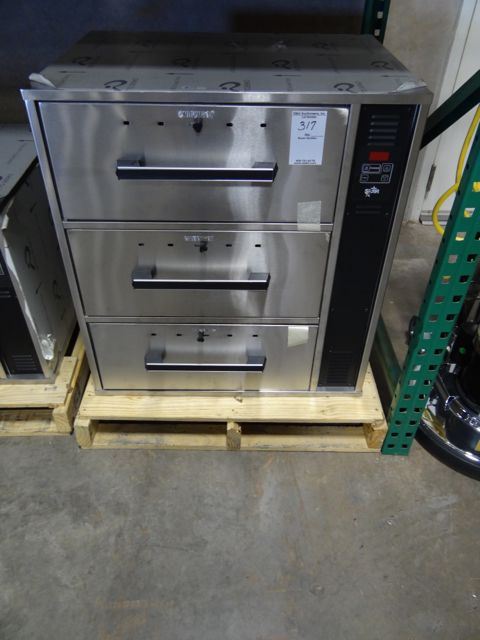The photograph shows a section of an indoor space, likely a warehouse, featuring a gray cement floor with scattered brownish dirt. In the background, the edge of a white door is visible at the top right corner. Next to the door, there is a green metal shelf frame containing two wooden pallets. The wooden pallet on the left holds a smaller metal device, similar to the main object but shorter.

In the foreground, the centerpiece of the image is a metallic appliance placed on a light brown, unfinished wooden pallet. This appliance resembles a metal filing cabinet with three large drawers, each equipped with blackish-silver handles. The top drawer has a protective sticker sheet, and a sticker with the date "3-7" on it. There is also a tall, black rectangular interactive panel with a red readout to the side of the drawers. The background shows the green metal frame of the shelf and another smaller version of the silver appliance partially cut off at the left edge of the image.